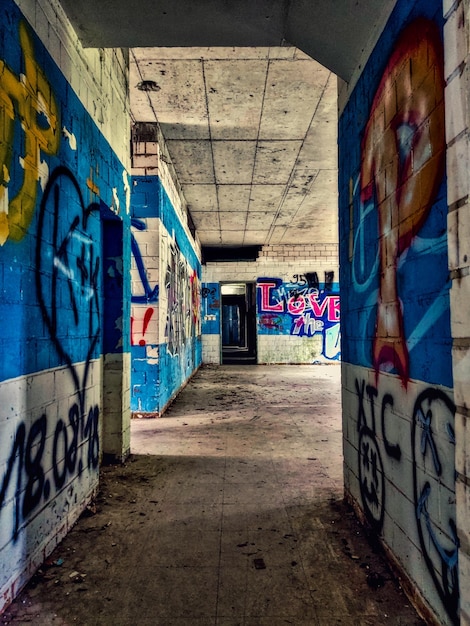This vertical rectangular photograph appears to be taken inside a decrepit or abandoned building, possibly a basement or under train tracks. The setting resembles a corridor leading to a larger, brighter room. The walls on each side of the corridor are coated in white and blue paint, with significant wear and dirt, indicative of decay. The floors and tiled ceiling share the gray, grimy state of disrepair. The corridor walls are heavily adorned with varied graffiti, displaying a predominant blue background with gold figures, and writings in black, yellow, and brown. Notably, on the right side of the doorway at the end of the corridor, bold red letters spell out "LOVE." Straight ahead, the larger room's far wall is also covered with blue-based graffiti and features a black heart inscribed with "K and K" and another message in pink letters with a white and purple outline stating "LOVE." Additional graffiti includes "1.8.08.18," "XTC," and emotive symbols like a smiley face with X's for eyes and a red exclamation point. The scene exudes both abandonment and an explosion of unauthorized art, capturing a raw, neglected beauty.